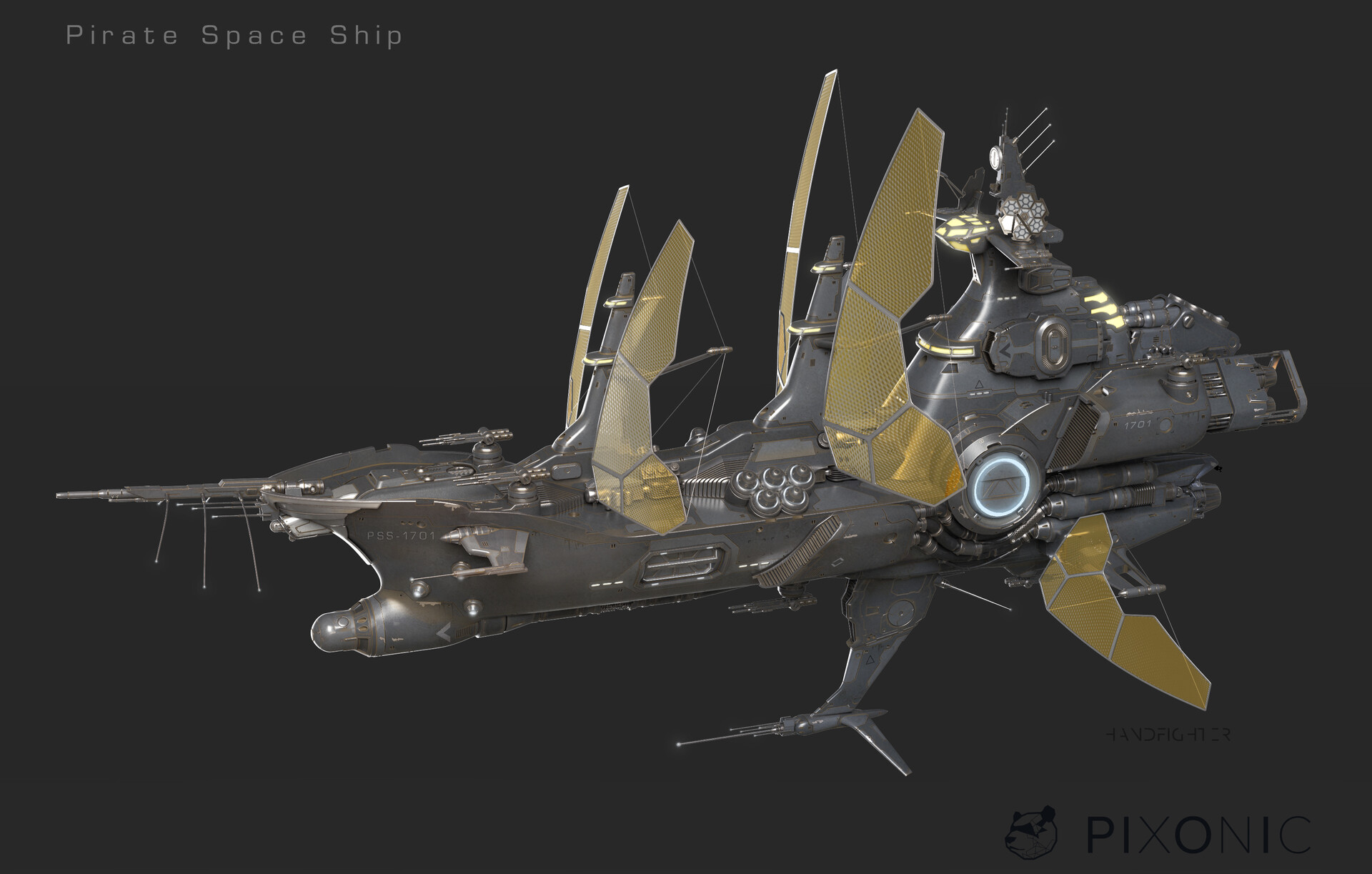The image is a highly detailed, computer-generated illustration of a futuristic pirate spaceship, reminiscent of designs from video games. The spaceship is prominently positioned in the center of a dark gray background, with the bow (front) oriented towards the left. The upper left corner of the image features the text "Pirate Spaceship" in a light grey or white font, while the lower right corner contains the text "Pia Xenus" along with a small panda logo. The spaceship itself exhibits a complex design, merging elements of traditional naval ships with advanced, sci-fi components. It has a rounded, grey hull with various extensions on the top and bottom that resemble a mix of sails and weapons. The sails are particularly distinctive, with transparent, see-through yellow sections supported by a grey outer edge and crisscrossing grid-like supports. The spaceship also features large guns, visible on both the bottom and the top, and the rear half of the ship resembles a spacecraft, complete with a control tower and what appears to be a large circular structure emitting a blue illumination. Additional features include various tubes, mechanical devices, and a grid pattern that suggests the presence of engines or other propulsion systems.

In summary, the image portrays an elaborate, 3D-rendered pirate spaceship combining futuristic and naval elements, set against a dark backdrop with specific text details in the corners.